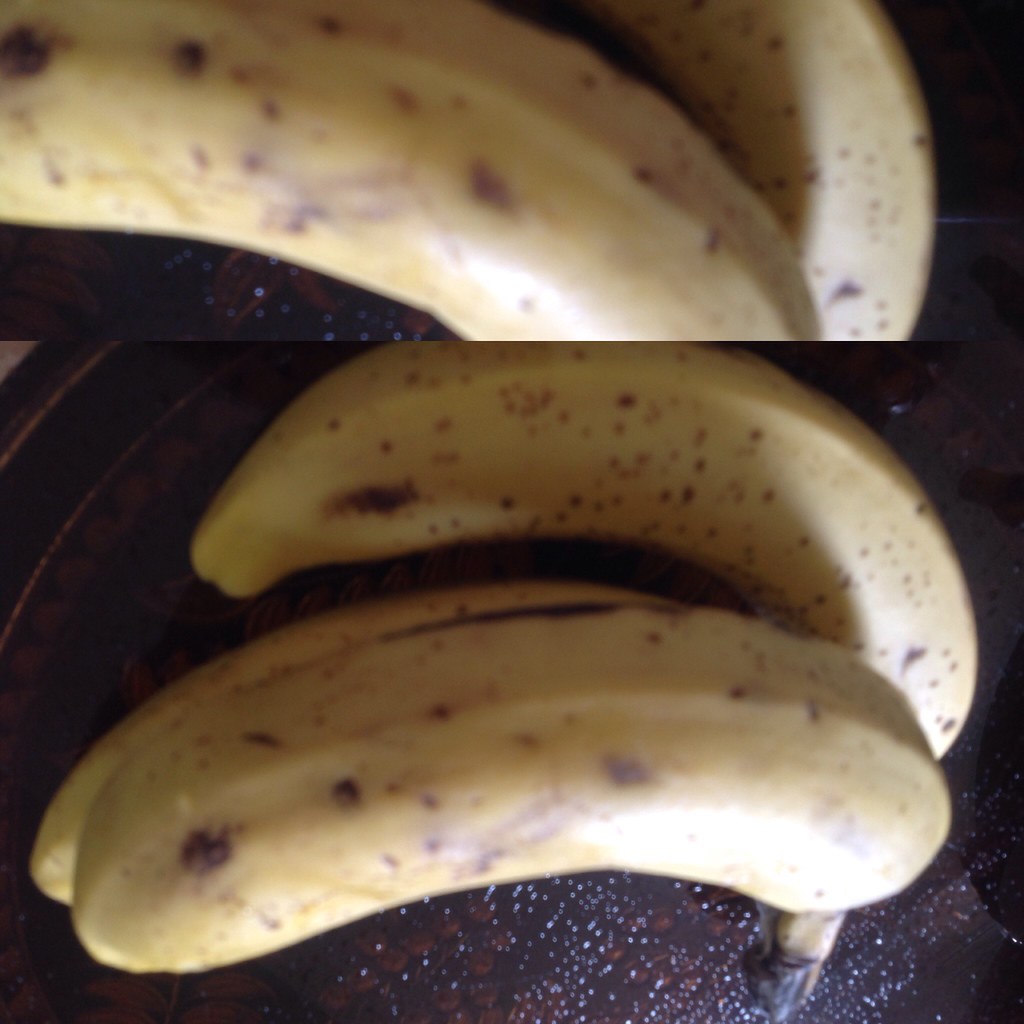The image consists of two closely cropped photos of bananas set against a purple-toned surface with bright, scattered dots. The top photo, taking up one-third of the overall image, provides an ultra-close, slightly blurry view of two bananas that are halfway ripe, starting to turn brown with small brown spots on their yellow peels. The very tip of one banana appears almost black. The bottom photo displays the same bananas at a slightly further distance, revealing medium-length bananas with a more detailed view of their natural blemishes. The bananas are resting in a tray, possibly brown, though it's not clearly visible, and there appears to be some reflection creating an illusion of more bananas. There is no text or words present in the image.